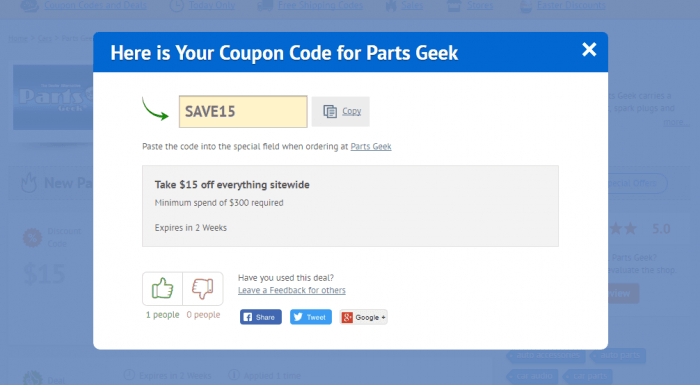The image is a screenshot featuring a coupon code for PartsGeek, showcased in a rectangular layout. The background of the image is a medium blue rectangle. Overlaid on this, there is a white rectangle with a bright blue header. The text within the header reads, "Here is your coupon code for PartsGeek" in white lettering, and a white 'X' for closing the window is located on the right-hand side of the header.

Beneath the header, a thin green arrow swoops down and points toward a yellow box. The yellow box contains the text "SAVE 15" in black, all capital letters, with a "Copy" button to its right.

Further down, the instructions "Paste the code onto the special field when ordering at PartsGeek" appear, with "PartsGeek" functioning as a clickable link. 

Following this, in a light gray box with bold lettering, the text announces, "Take $15 off everything site-wide." Additional fine print below, in medium gray, mentions, "Minimum spend of $300 required," and "Expires in two weeks."

Returning to the white background below the gray box, there are feedback options showing one person has given a thumbs up, while no one has given a thumbs down. A small black text queries, "Have you used this deal?" directly above a blue underlined link prompting, "Leave a feedback for others." At the bottom, options to share the deal are provided via buttons for Facebook, Twitter, and Google Plus.